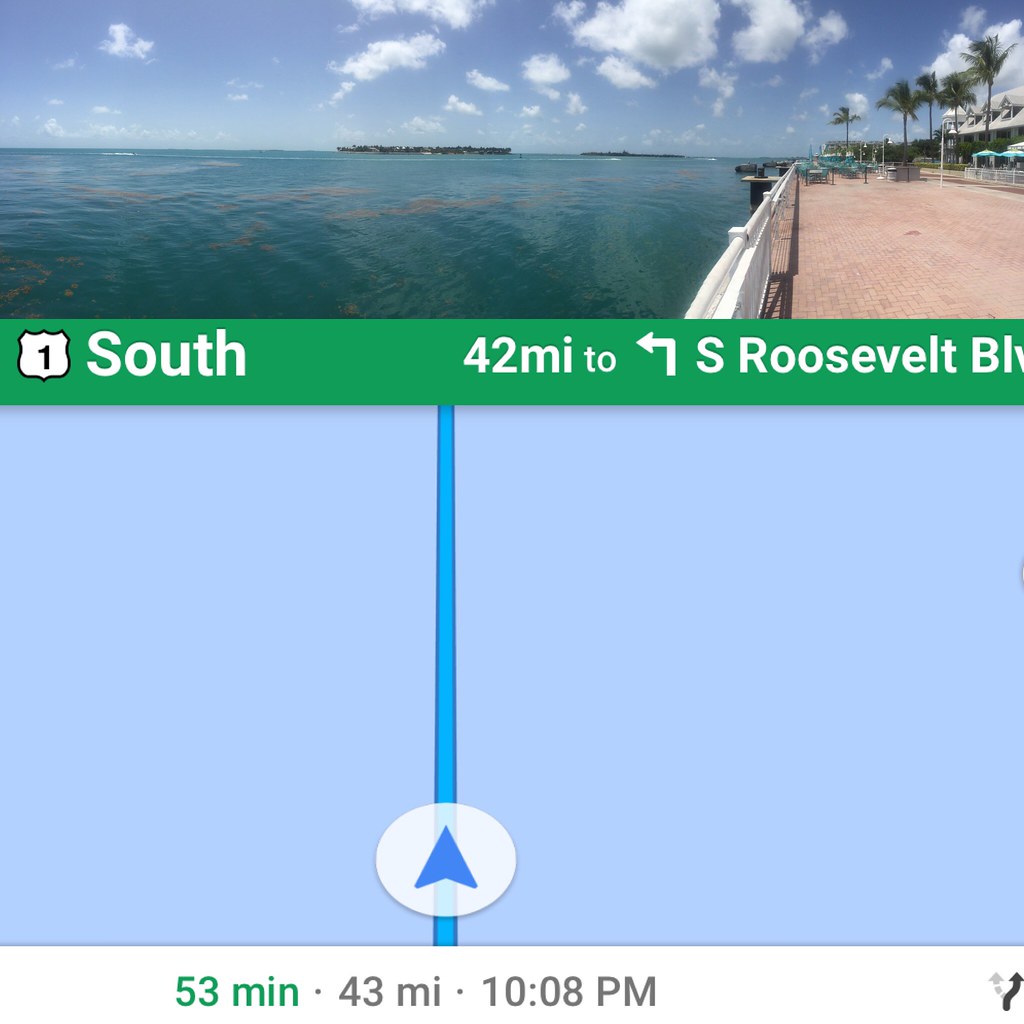This image appears to be a navigation screenshot, possibly from MapQuest, Waze, or Apple Maps, providing driving directions. The center of the image prominently displays a map with a light blue background, featuring a vertical bright blue line and a blue arrow encompassed in a white circle, indicating the car's current path. A green banner in the middle of the screen reads "South 42MI to left arrow S Roosevelt BLVD" with highway symbol numerals "1" and "South" in white text. The navigation indicates that the route is on Highway 1 South for 42 miles, with an expected left turn onto South Roosevelt Boulevard.

At the top third of the image, there is a captivating photograph depicting a serene ocean scene with two small islands in the distance. A beautiful brick walkway runs alongside the calming blue waters, bordered by a white fence. The picturesque view also includes palm trees, turquoise chairs, and an area with umbrellas suggesting a nearby hospitality venue, possibly a hotel or beachfront restaurant. This scenic destination is detailed further with a serene blue sky dotted with white puffy clouds, enhancing the tranquil and inviting atmosphere.

The overall route is a distance of 43 miles, taking approximately 53 minutes to drive, with an anticipated arrival time of 10:08 PM.